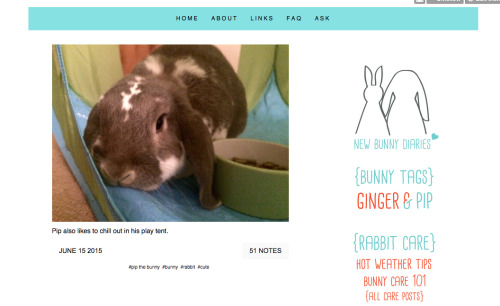The website features a prominently displayed image of two bunnies. The first bunny is brown with a distinctive white line running from between its eyes to the back of its head, accompanied by additional white markings on its back and cheeks. The bunny is resting its head on what appears to be a blue mat. Positioned next to the bunny is a small green bowl containing food. 

Above the image, there is a turquoise navigation bar with various menu options including: Home, About, Lines, Facts, Ask, Bunny Tags, Ginger and Pep, Rabbit Care, Hot Weather Tips, and Bunny Core Care 101.

Beneath the image, a caption reads: "Pip also likes to chill out in his playland." To the right of the caption is a date stamp and an indication that the post has 51 notes. The entire webpage is set against a clean, white background.